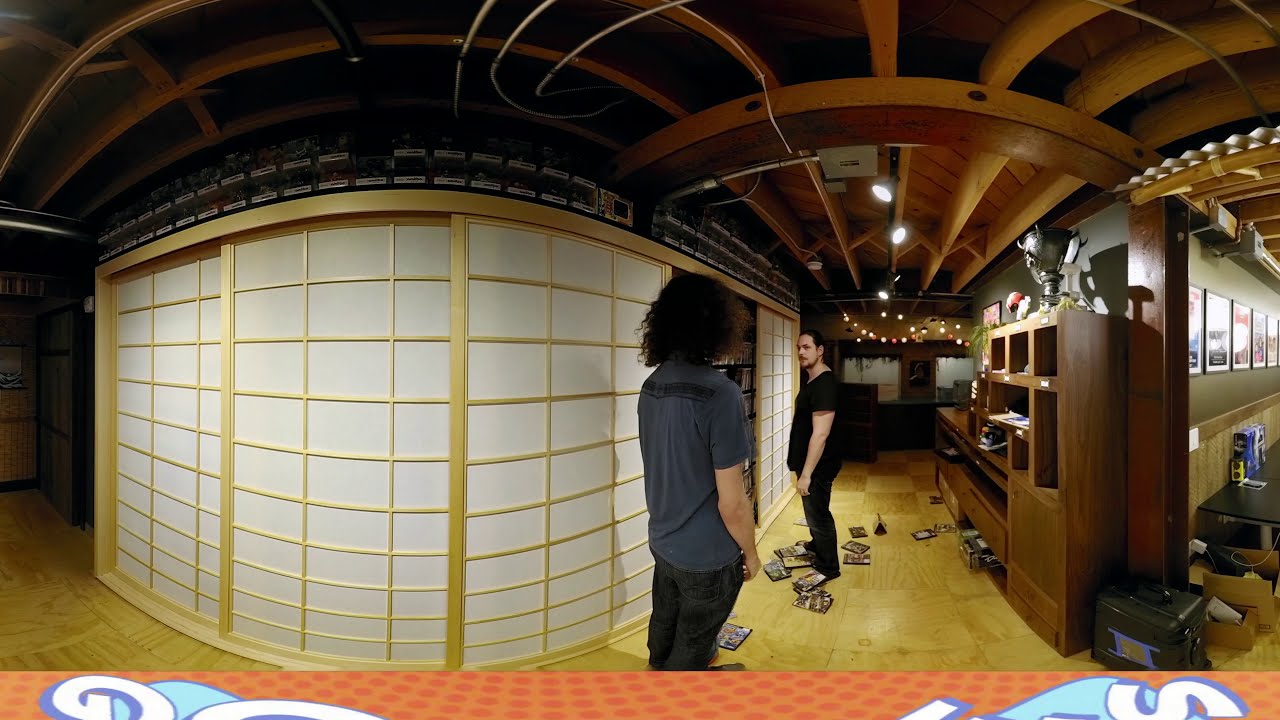The image captures a detailed scene inside a bright, possibly modern office space with elements resembling a home. Two men are standing in a three-quarter turn towards each other in a hallway, with contrasting appearances. The man facing away from the camera has shoulder-length frizzy, dark curly hair, is wearing a blue shirt and dark gray pants. The other man, facing towards the camera, is characterized by a mustache and beard, donning a black shirt and pants. They are positioned inside a room with a fishbowl-like perspective that gives a slightly rounded view.

The environment features a distinctive white awning with light wood frames creating a checker pattern across the door, and a wooden ceiling with prominent beams. The floor has a yellowish-tan hue, and to the right, brown bookshelves are evident, along with a large dresser and scattered cases on the floor. A prominent trophy is noticeable atop the hallway, leading towards another room.

In the foreground, there is a logo with partially visible letters “G” and “S” on an orange background with red dots, situated in front of a Japanese-style partition. This combination of delicate features and clutter suggests a nuanced mix of residential and commercial design, further emphasized by seating arrangements and picture frames on the wall indicative of a restaurant-like setting. Overall, the vibrant colors and intricate details create a rich, dynamic atmosphere.